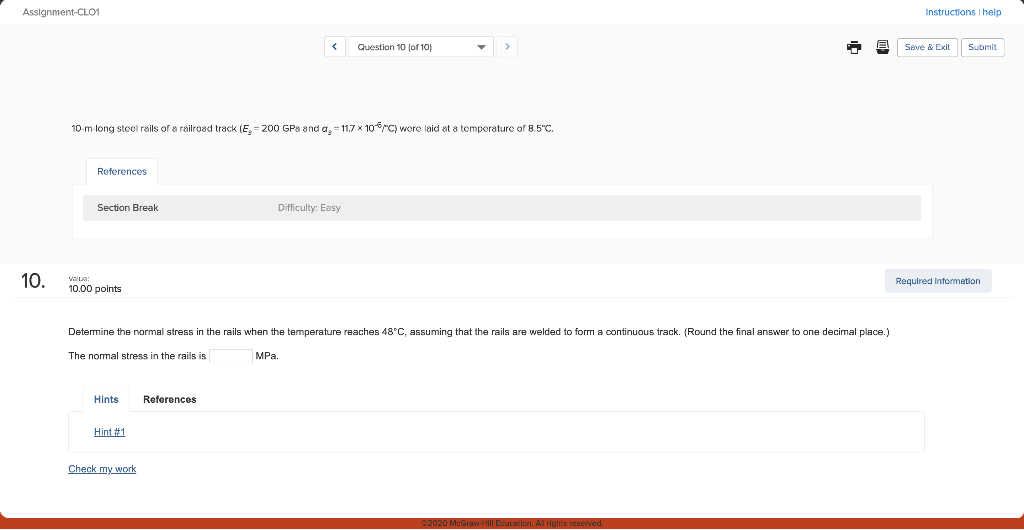In this detailed screenshot of a website with a white background, various elements can be observed. In the upper left-hand corner, there is the text "assignment-CLO1." On the upper right-hand corner, two hyperlinks labeled "Instructions" and "Help" are visible. 

Centrally located, the page displays "Question 10 of 10" prominently, along with adjacent arrow toggles that allow navigation between questions, and a drop-down arrow for additional options. Below this, there are icons for printing the page, signified by a printer graphic, and buttons for "Save and Exit" and "Submit," which are presented as rectangular buttons accompanied by blue hyperlink text.

The main section contains a mathematical question regarding "10-millimeter long rails of a railroad track," including an equation to be solved. Just after the question, there is a section break followed by the tag "Difficulty" which states that the question is categorized as "Easy." Further, it notes that this particular question, number 10, is worth 10,000 points. Additional interactive elements include a "Hints" button, a "Check My Work" button, and a "Required Information" button, providing various levels of assistance for the user.